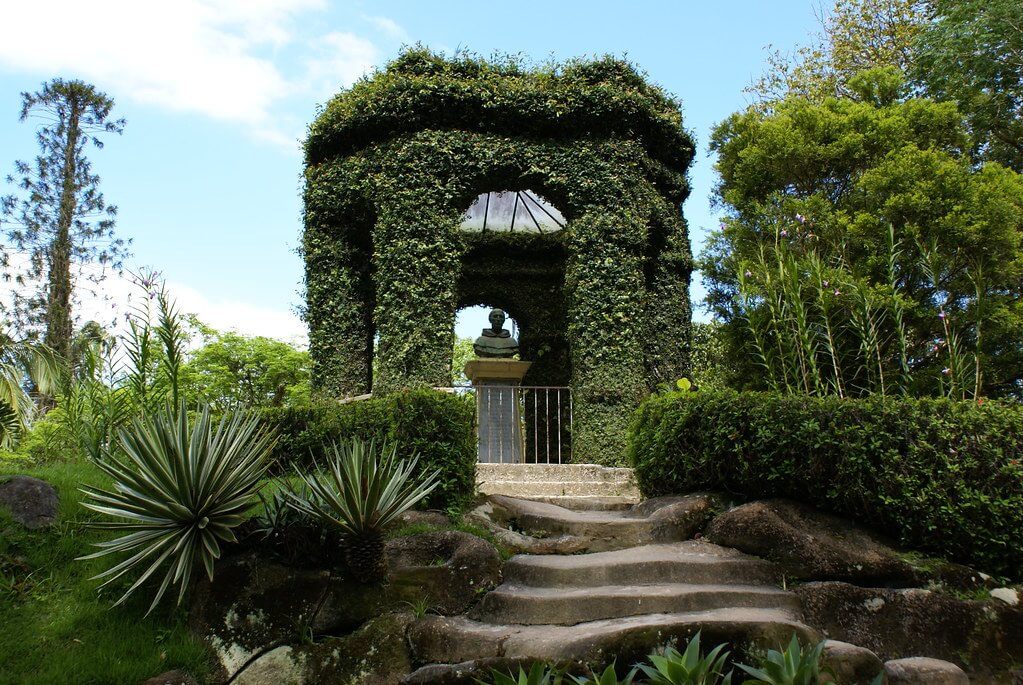The photo captures a meticulously manicured outdoor garden estate featuring a prominent gazebo structure covered with lush ivy and green leaves. The gazebo, which has a glass skylight free of vegetation and a curved roof, stands elevated on weathered stone steps and is surrounded by a silver metal gate. In the center of the gazebo, there is a bust of a man on a pedestal, possibly a religious or culturally significant statue. Leading up to the gazebo, stone steps and a wooden path wind through the vibrant garden. The garden is filled with various types of greenery, including manicured hedges, spiky plants, and a range of other flowering plants. To the left, a towering tree with dense foliage crowns over sparser vegetation, while on the right, a dense collection of tall trees marks the garden's edge. The bright blue sky above is mostly clear, punctuated by wisps of white clouds, while the sun’s position creates a slight overexposure in the top left corner of the image. Overall, the scene is tranquil and well-maintained, invoking a sense of serene beauty.